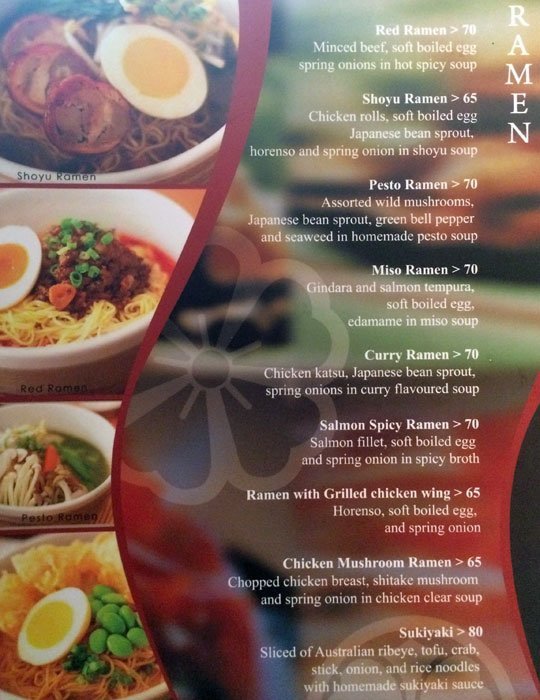This image is a detailed menu page from an Asian restaurant, showcasing a variety of ramen dishes. The left side features four full-color photos of ramen bowls, including Red Ramen, Shoyu Ramen, and Pesto Ramen, while the bottom picture is unlabeled. Marking a distinction, a red swooping border separates these images from the dish names and prices on the right. Each ramen is tagged with its unique price and description, all written in white text. Starting from the top of the list, the dishes and ingredients are meticulously outlined: Red Ramen with minced beef, soft-boiled egg, spring onions, and hot spicy soup ($70); Shoyu Ramen with chicken rolls, soft-boiled egg, Japanese bean sprout, horenso, and spring onion in shoyu soup ($65); Pesto Ramen featuring assorted wild mushrooms, Japanese bean sprout, green bell pepper, and seaweed in homemade pesto soup ($70); Miso Ramen with jindera and salmon tempura, soft-boiled egg, edamame in miso soup ($70); Curry Ramen with spring katsu, Japanese bean sprout, spring onions, and curry flavored soup ($70); Salmon Spicy Ramen with salmon filet, soft-boiled egg, and spring onion in spicy broth ($70); Ramen with Grilled Chicken Wing, horenso, soft-boiled egg, and spring onion ($65); Chicken Mushroom Ramen with chopped chicken breast, shiitake mushrooms, and spring onion in clear chicken soup ($65); and Sukiyaki with sliced Australian ribeye, tofu, crab stick, onion, and rice noodles in homemade sukiyaki sauce ($80). The background is a multicolored design without clear definitions, adding a vibrant flair to the presentation.